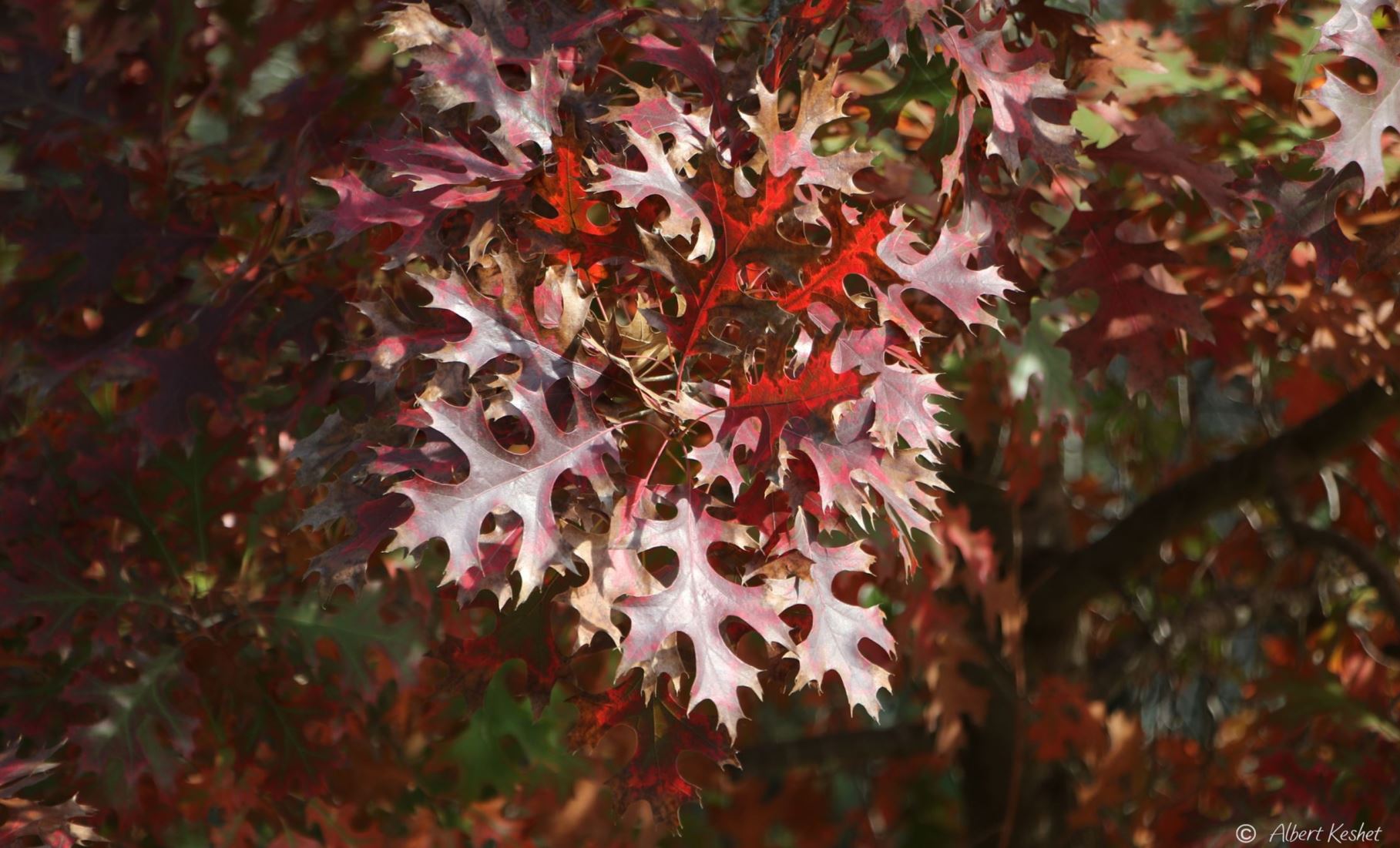This image captures a close-up view of a cluster of leaves during the fall, emphasizing their intricate structure and vivid autumn colors. The photograph, credited to Albert Keshet, centers on a symmetrically arranged bunch of narrow, pointed leaves, each stemming from a central vein and branching out into three sections that converge at the tip. These leaves display a striking palette of reds, oranges, and browns, indicative of the seasonal change, while their undersides appear almost whitish. The background is a blur of additional foliage, with hints of a tree trunk and larger branches partially visible, enhancing the focus on the foreground leaves. This blurring technique sharpens the central leaves, making it clear they are the main subject of the photograph. The scene depicts a mix of leaf colors, including some green, suggesting a transitional period in fall where the outer leaves exposed to sunlight turn red first while the more sheltered ones retain some green.